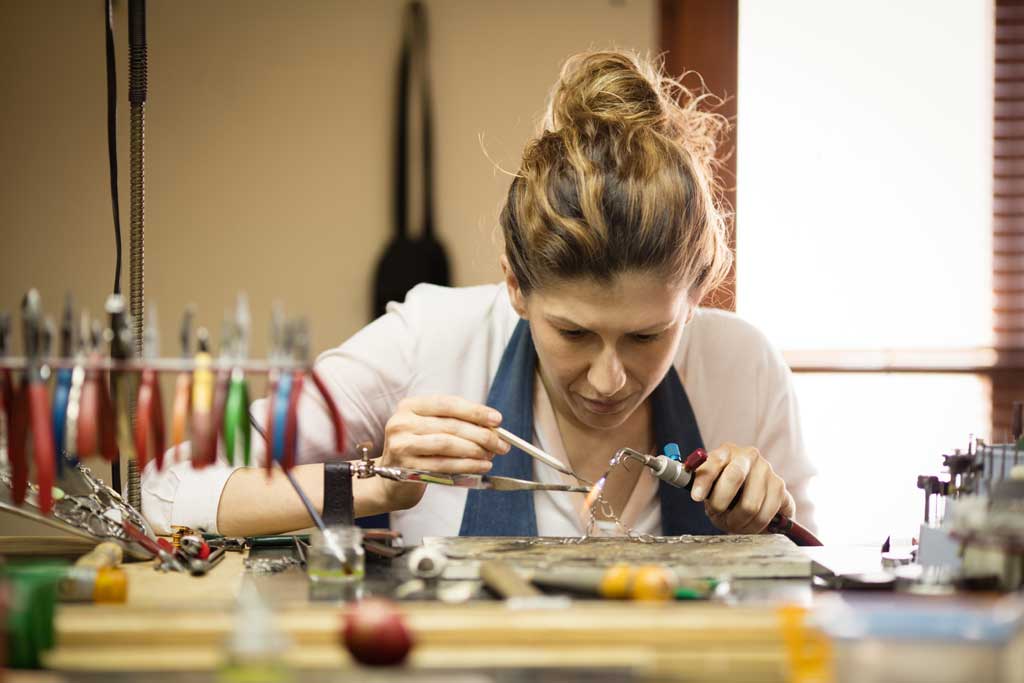The photograph captures a young woman deeply engrossed in her work in a workshop setting. She has her brown, highlighted hair pulled back into a messy bun and is wearing a white shirt paired with a blue apron or vest. She is seated at a cluttered tabletop, visible from the chest up, leaning over a piece of metal or jewelry. In her left hand, she holds a small handheld welding tool emitting a spark, while her right hand is equipped with what appears to be a tweezer or pick, indicating she is meticulously assembling or welding something. The table in front of her is strewn with various tools, including a bar on the left side that holds pliers of multiple colors—red, green, blue, yellow, and orange. The background features a blurry beige wall and a large window on the right, but the focus remains sharply on her concentrated expression and precise movements.